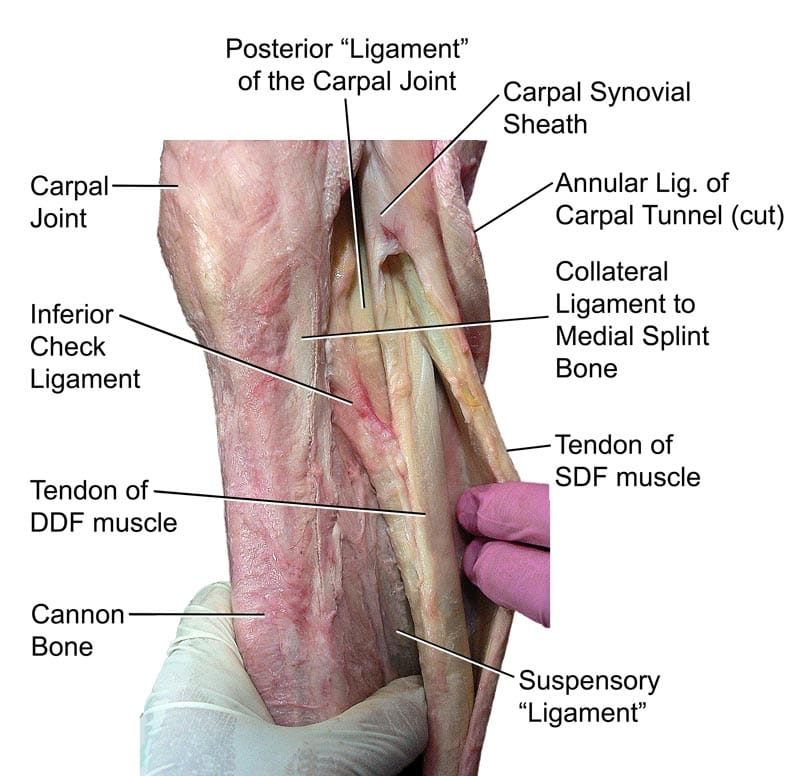This detailed image, likely from an anatomy and physiology textbook, provides a close-up view of various structures in the arm, specifically focusing on the carpal joint and its associated muscles, tendons, and ligaments. The picture is annotated with extensive black text labeling each anatomical feature. The primary structures identified include the posterior ligament of the carpal joint located at the top, the carpal synovial sheath to its right in the upper right-hand corner, and the annular ligament of the carpal tunnel, which is cut. Additional labels point to the collateral ligament to the medial splint bone, the tendon of the SDF muscle, the suspensory ligament at the bottom right, and the cannon bone at the bottom left. To the left, the tendon of the DDF muscle and the inferior check ligament are indicated, with the carpal joint appearing in the top left-hand corner. The hands handling the specimen are wearing surgical gloves; the right hand sports a pink glove, while the left hand is gloved in green. This comprehensive labeling provides a detailed educational reference for understanding the intricate components of the carpal joint and surrounding tissues.